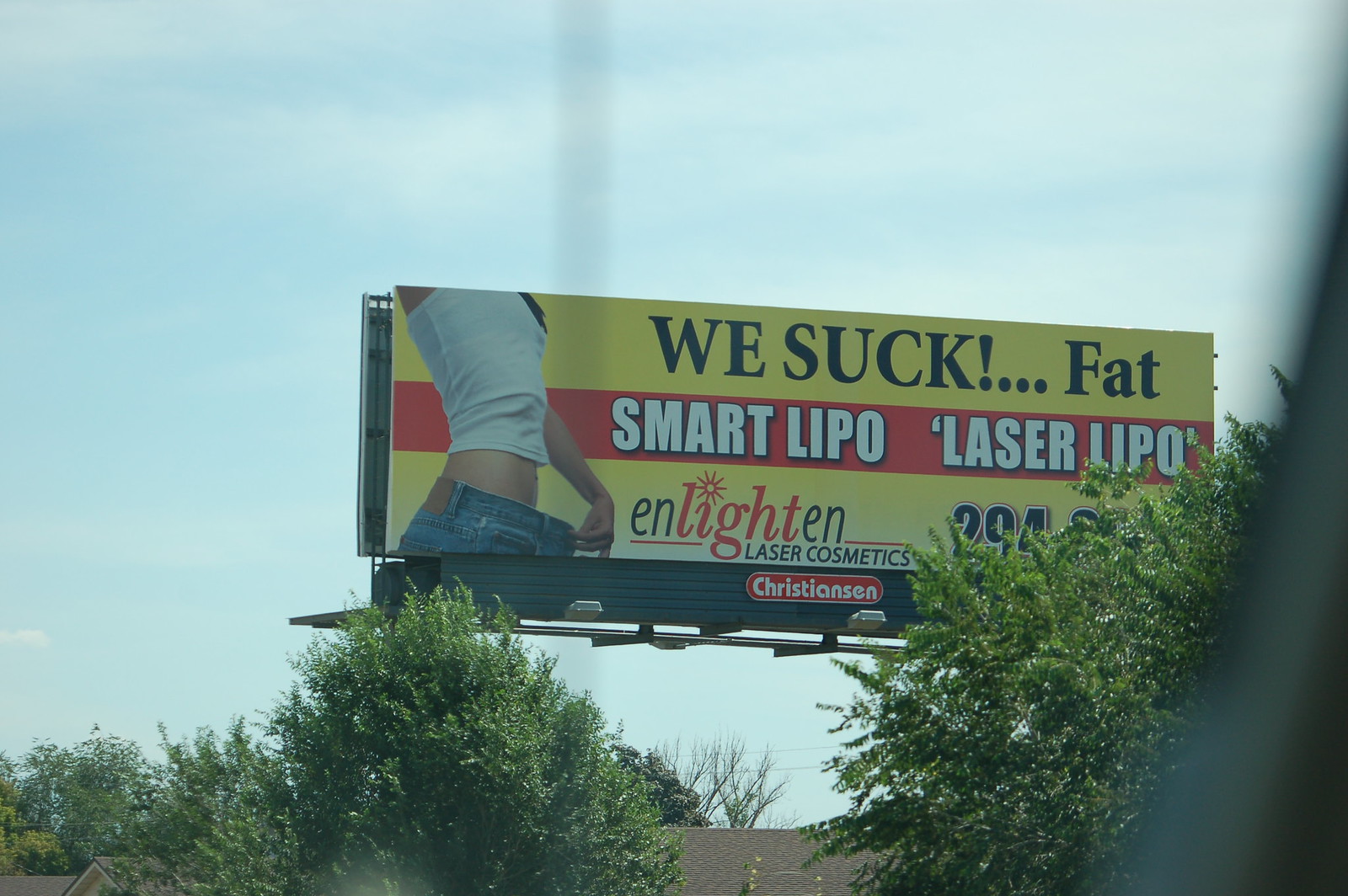This is a detailed description of a billboard advertising a cosmetic procedure:

The large billboard prominently features a bold, eye-catching yellow background with the stark black letters "WE SUCK FAT" displayed at the top. The central image showcases a woman demonstrating her slim figure by pulling out her loose-fitting jeans away from her belly, though only the middle portion of her body and the one arm holding the pants are visible. Dividing the billboard vertically, a red stripe reads "Smart Lipo Laser Lipo," while "Enlighten Laser Cosmetics" is printed below it. A phone number is situated on the lower right side, nearly hidden by the greenery from a nearby tree. The billboard is branded with the name "Christiansen" located discreetly in the corner. The surrounding area features additional greenery and shrubs, along with the visible top roof of a house in the background, contributing to the suburban setting.